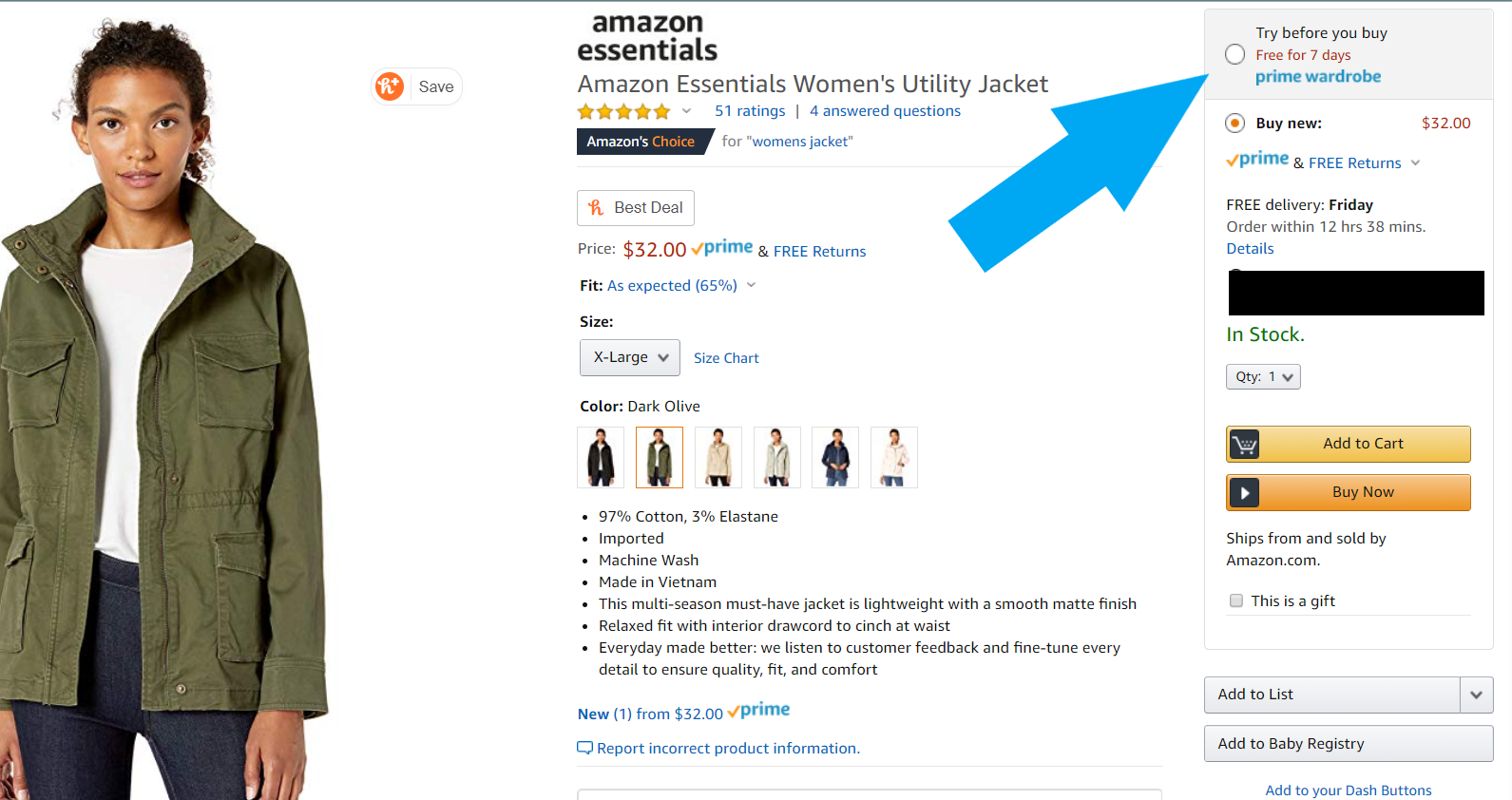**Descriptive Caption for the Amazon Product Image:**

The image depicts a screenshot from the Amazon website, showcasing a product listing for the 'Amazon Essentials Women's Utility Jacket.' The focal point of the image is a young African-American woman in her early 30s standing to the left. She has slightly messy hair pulled back into a ponytail with some strands sticking out. She wears a modest smile, a floral green jacket over a white shirt, and dark blue jeans.

To her right is the product information on a clean, white background. The jacket is identified as an 'Amazon Essentials Women's Utility Jacket,' adorned with a 5-star rating based on 51 reviews and 4 answered questions. Additionally, it features the 'Amazon's Choice' label, highlighting it as a top pick in women's jackets.

The jacket is priced at $32 with the benefits of Amazon Prime, including free returns. A note indicates that 65% of customers found the fit as expected. The selected size displayed is XL (extra-large), and a size chart is available for reference. The highlighted color is dark olive, but six thumbnails show the jacket in other colors: black, dark olive, beige, light gray, navy blue, and white.

Product details specify that the jacket is made of 57% cotton and 3% elastane, imported, machine washable, and manufactured in Vietnam. It is designed for multi-season use, with a lightweight and smooth finish, constructed for a relaxed fit that accentuates the waist. The product aims for enhanced quality, fit, and comfort based on customer feedback.

The right side of the image features a prominent blue arrow labeled 'Try before you buy,' offering a 7-day free trial under Prime Wardrobe or the option to purchase the jacket outright for $32. Delivery estimates suggest arrival by Friday if ordered within 12 hours and 38 minutes.

Below, an 'In Stock' notice is highlighted, with a default quantity of one. There are options to 'Add to Cart' or 'Buy Now,' with shipping and selling managed by Amazon. Additional features include a checkbox to mark the item as a gift and options to add the jacket to a list, baby registry, or Dash button.